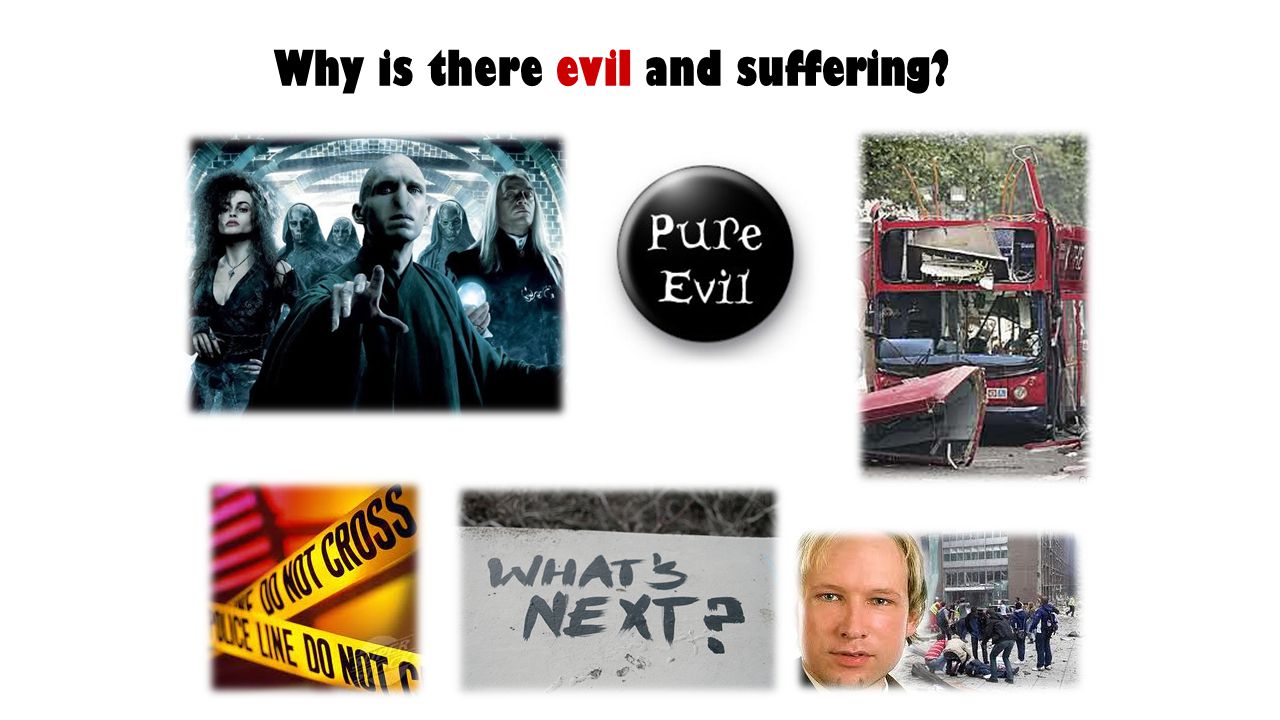The image is a detailed collage, featuring a mix of six distinct pictures arranged in two rows against a pure white background, resembling a PowerPoint presentation. At the very top, a bold text, "Why is there evil and suffering?" is displayed, with the word "evil" highlighted in red while the rest is in black font. 

Starting from the top left, the first image depicts Voldemort and his Death Eaters from Harry Potter, resembling a movie cover. To the right of this, there's a black button with "Pure Evil" inscribed in white font. The third image in the top row showcases a destroyed double-decker bus, indicative of a severe accident.

In the bottom row, the far left image shows police "Do Not Cross" tape stretched across a red background. Next to it, there's a white sign with "What's next?" written in black marker. The final image on the bottom right captures a chaotic scene involving several people gathered around someone on the ground, with a close-up of a blonde man with blue eyes staring intensely.

The overall composition employs colors such as black, white, red, various shades of blue, pink, purple, green, and gray, amplifying the sense of disorder and emphasizing the theme of evil and suffering.